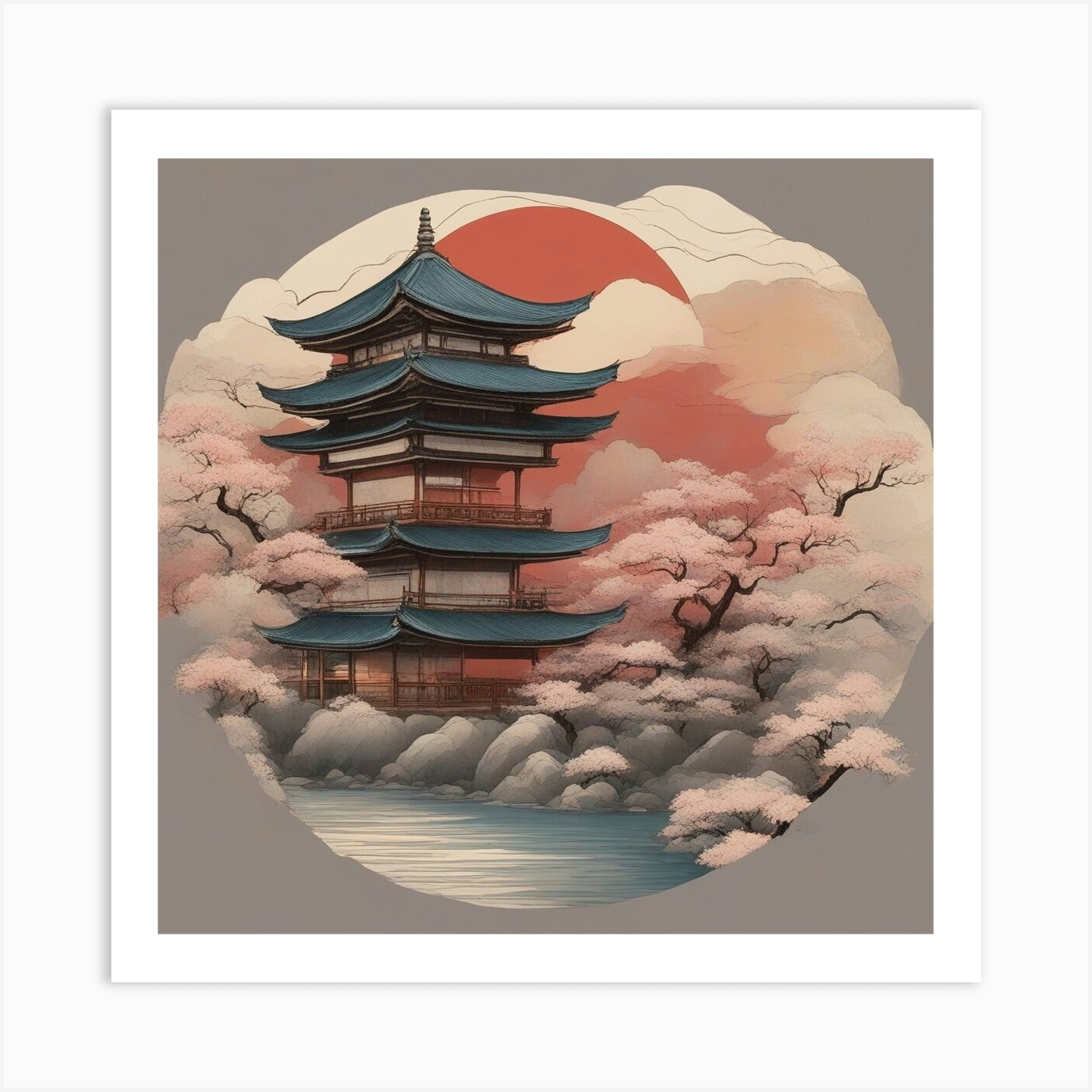This is a detailed photograph of a painting that captures a traditional Edo Japanese castle with four visible levels at its center. The castle features gray-blue roofs and wooden banisters around two of its stories, set against beige-gray and darker gray backgrounds. The lower portion of the castle appears larger than the upper levels, with white walls accented by brown. Surrounding the castle at its base are multiple rocks and cherry blossom trees with vibrant pink leaves on both sides. A blue river with white streaks flows near the rocks. Above the castle, a salmon-colored sun—depicting either sunrise or dusk—is surrounded by circular, white-gray clouds with hints of orange and pink. The castle, river, and trees are all enclosed within a circular frame, beyond which lies a grayish expanse. The painting employs a kimono-style, silkscreen technique, with the predominant colors being pink, orange, and white.